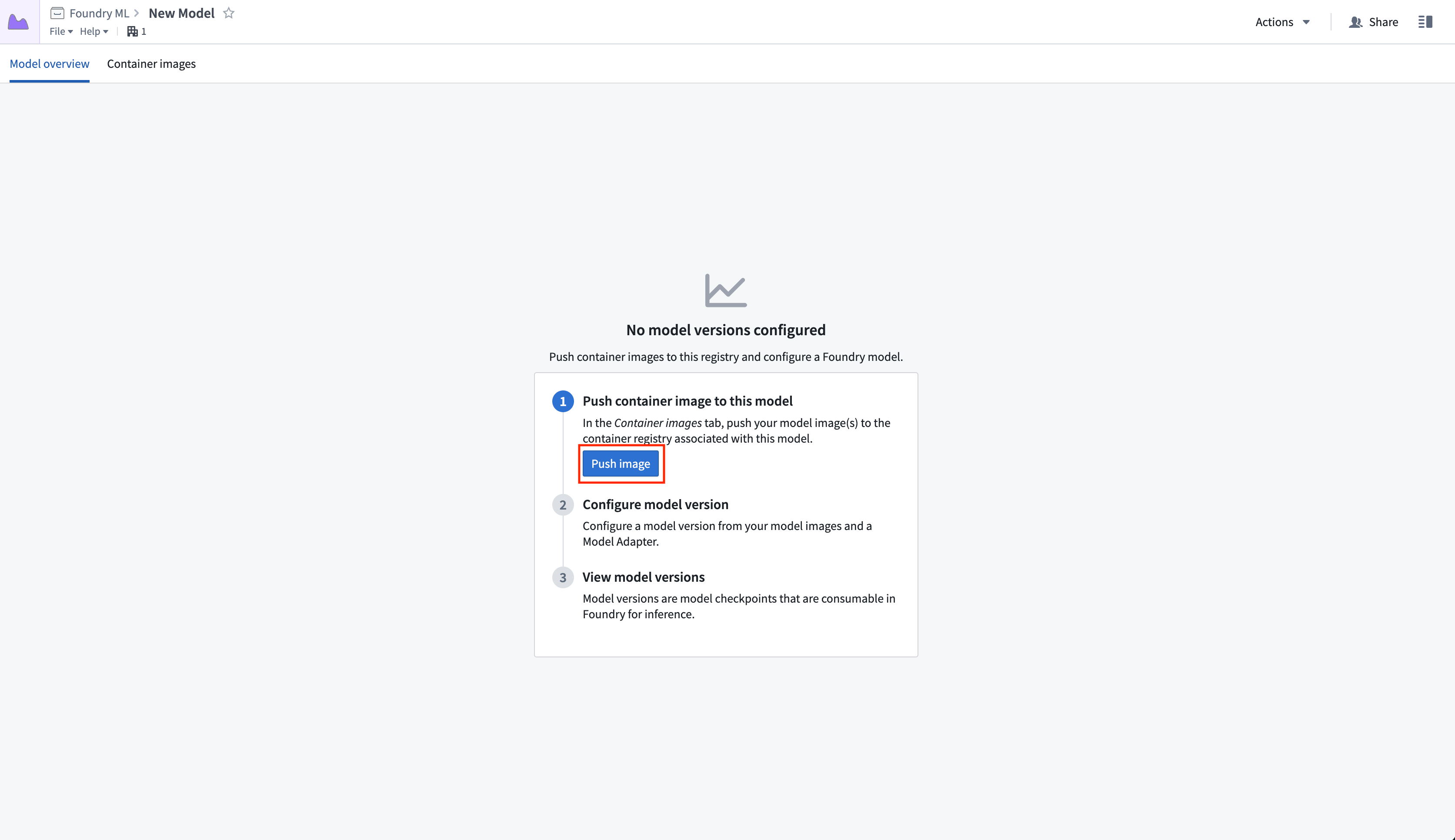This screenshot showcases a panel within the Foundry ML software, a machine learning platform designed for scientists. In the top left corner, "Foundry ML" is subtly displayed in small gray font. An arrow pointing to the right leads to "A New Model," prominently featured in bold, small black font, accompanied by an unclicked star icon. 

On the top right, a dropdown box labeled "Admin" is visible, adjacent to a "Share" button. Below, on the left side, the navigation menu highlights "Model Overview" in light blue, juxtaposed with "Container Images" to the right. The "Model Overview" option is currently selected.

The main body of the page has a gray background. Centrally located, there is a message in small black font stating, "No model versions configured." Underneath this message, a white box is presented, which outlines three vertical steps for the user:

1. **Push container image to this model** - followed by a brief description.
2. The corresponding blue button labeled "Push Image" is accentuated with a red box, indicating a prompt for user action.

This scene effectively details the interface layout and user guidance elements within the Foundry ML platform, emphasizing the steps necessary to configure a new model.